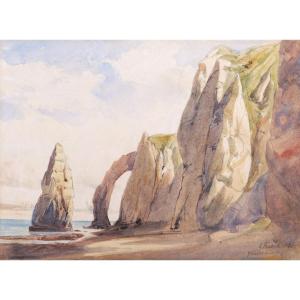This detailed hand-painted beach scene, possibly rendered with watercolor or soft pastels, captures a serene coastal landscape. The backdrop features a sky blending light blue shades with fluffy white clouds, setting a tranquil mood despite the overcast day. Majestic rock formations rise prominently from the sandy beige to darker brown beach and out of the water, showcasing a harmonious mix of tan, greenish-yellow, dusty blue, and dusty red hues. Among these rocks, a notable triangular rock stands tall on the right, while another impressive archway structure emerges from the water, seamlessly connecting to cliff areas. The cliffs themselves, painted with accents of white and green, run along the right-hand side, creating a striking contrast against the soft pastel colors and gentle beach setting. The calm waters mirroring the sky complete this picturesque and tranquil coastal scene.